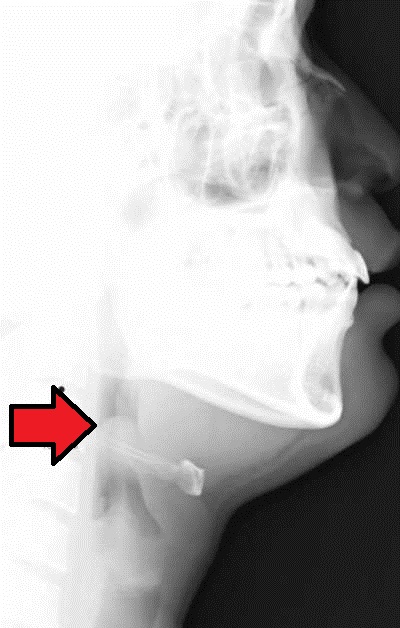The image depicts a detailed black and white x-ray of a person's side profile, spanning from the forehead to the top of the neck. The x-ray background is predominantly black, highlighting the skeletal structure, including the eye socket, nostril, mouth, teeth, jawline, and neck. A very large, thick red arrow is prominently placed on the left-hand side, pointing to a conspicuous object lodged sideways in the person’s throat, sticking out to the right. The person's mouth appears slightly open, further exposing the teeth and jaw area. The contrast in the x-ray emphasizes the delicate structures of the bones and the abnormality indicated by the arrow.